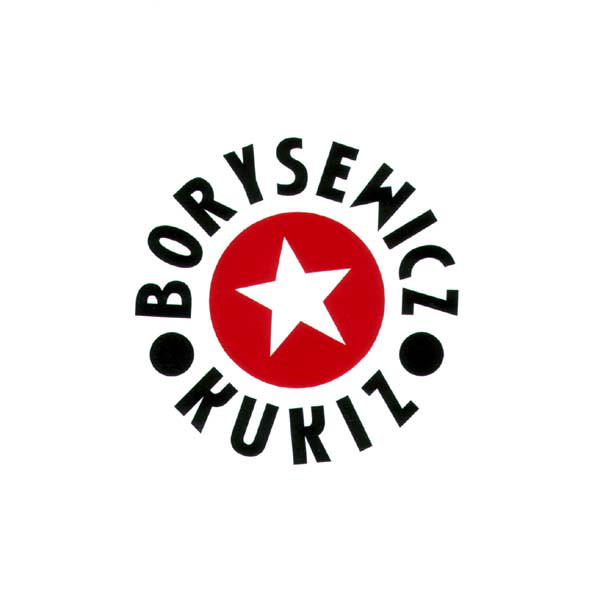The image displays a simple but detailed logo set against a white background. Dominating the center is a red circle featuring a slightly tilted five-pointed white star. Encircling this red circle, the word "BORYSEWICZ" is written in sharp, capital letters along the top, with two large black dots flanking the B and the Z. Mirroring this arc at the bottom of the red circle, the word "KUKIZ" in the same distinctive font completes the design. The overall composition of the letters and black dots forms a larger circular boundary around the red and white star emblem.